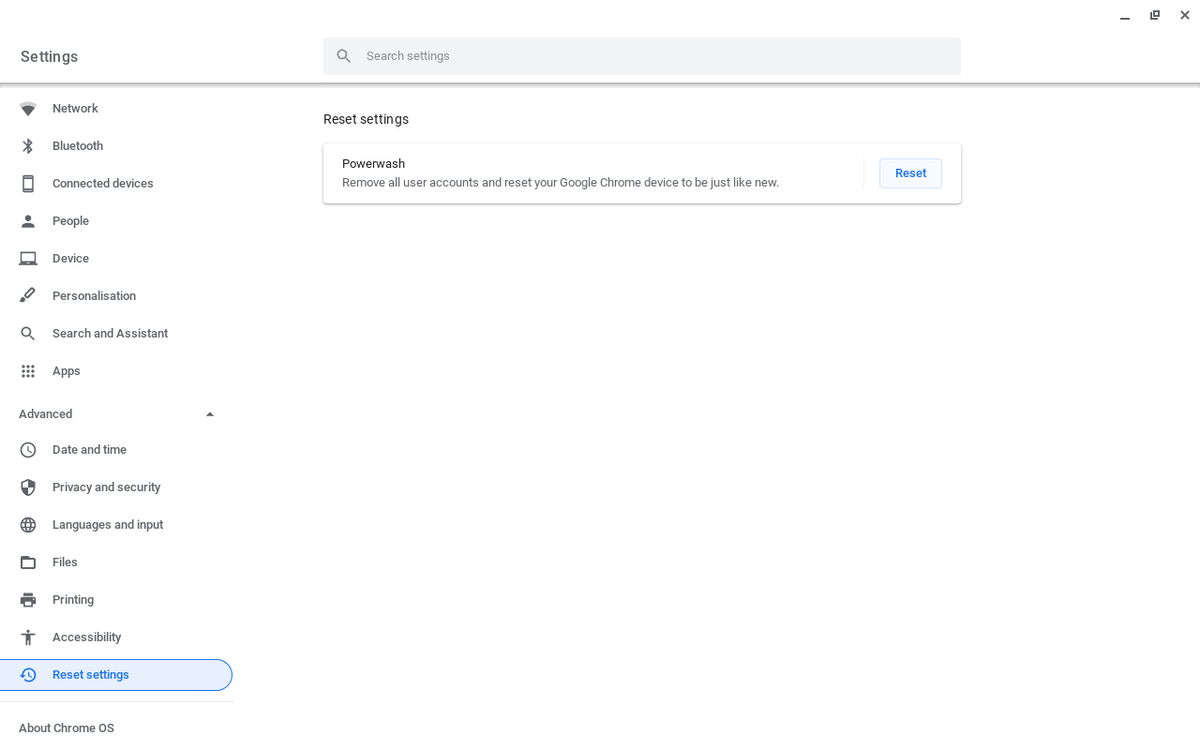This image is a detailed screenshot of the settings menu in Google Chrome OS, likely viewed on a computer or Chromebook. The menu displayed includes several prominent categories: Network, Bluetooth, Connected Devices, People, Device, Personalization, Search and Assistant, and Apps. Additionally, there is an "Advanced" section which encompasses more settings such as Date and Time, Privacy and Security, Languages and Input, Files, Printing, and Accessibility.

At the bottom of the menu, there is a section titled "About Chrome OS” next to which is located the “Reset settings” option. The user appears to have selected the "Reset settings" option, revealing further functionalities like "Powerwash." This feature allows the user to remove all user accounts and reset the Google Chrome device to its original, factory-like state. There's a noticeable blue "Reset" button associated with this option.

The screenshot highlights the practicality of the reset function, suggesting that it allows for a more efficient solution to clear all personal data and settings at once, rather than manually removing each account individually. This serves as a handy tool for anyone looking to completely refresh their device.